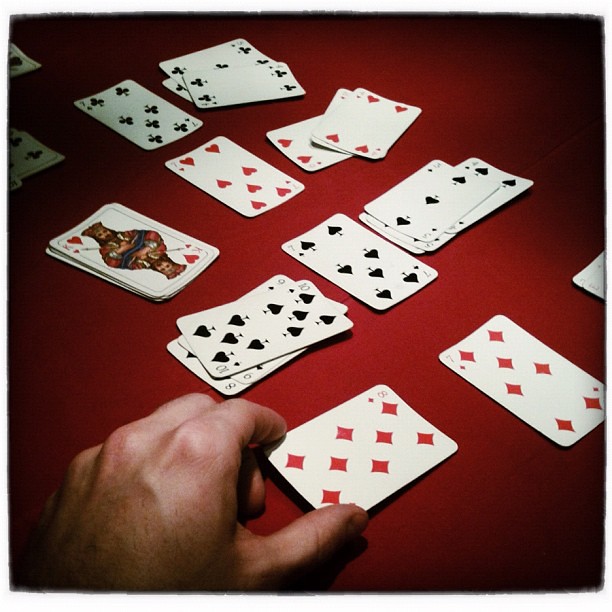The photograph captures an arrangement of playing cards meticulously laid out on a flat, red fabric-covered surface. The image has a square aspect ratio, with the longer sides being the left and right edges, giving it a composed yet dynamic feel. The borders of the image have been artistically edited to appear frayed and weathered, creating a grayed, aged look with various small chunks missing. The edges are heavily blackened, particularly in the bottom right, bottom left, top left, and top right corners, which adds a moody, almost vignette effect to the overall composition.

Emerging from the bottom left corner is a light-skinned human left hand, with fingers gracefully poised to pick up a playing card. The hand is delicately holding the 8 of Diamonds between the index finger and thumb. This card prominently features a large red number 8 in the top left corner and is decorated with eight diamond shapes arranged in a symmetric pattern. Adjacent to it is the 7 of Diamonds, easily identifiable by the red number 7 in the top left corner and seven red diamond shapes.

Several neatly stacked piles of cards are laid out beside the hand. To the left of the hand's position, a noticeable pile exclusively consists of cards from the suit of Spades, exhibiting multiple numbers from that suit. The careful positioning and selection of these elements bring a sense of anticipation and strategy inherent in a card game, all set against the rich, velvety red fabric backdrop.